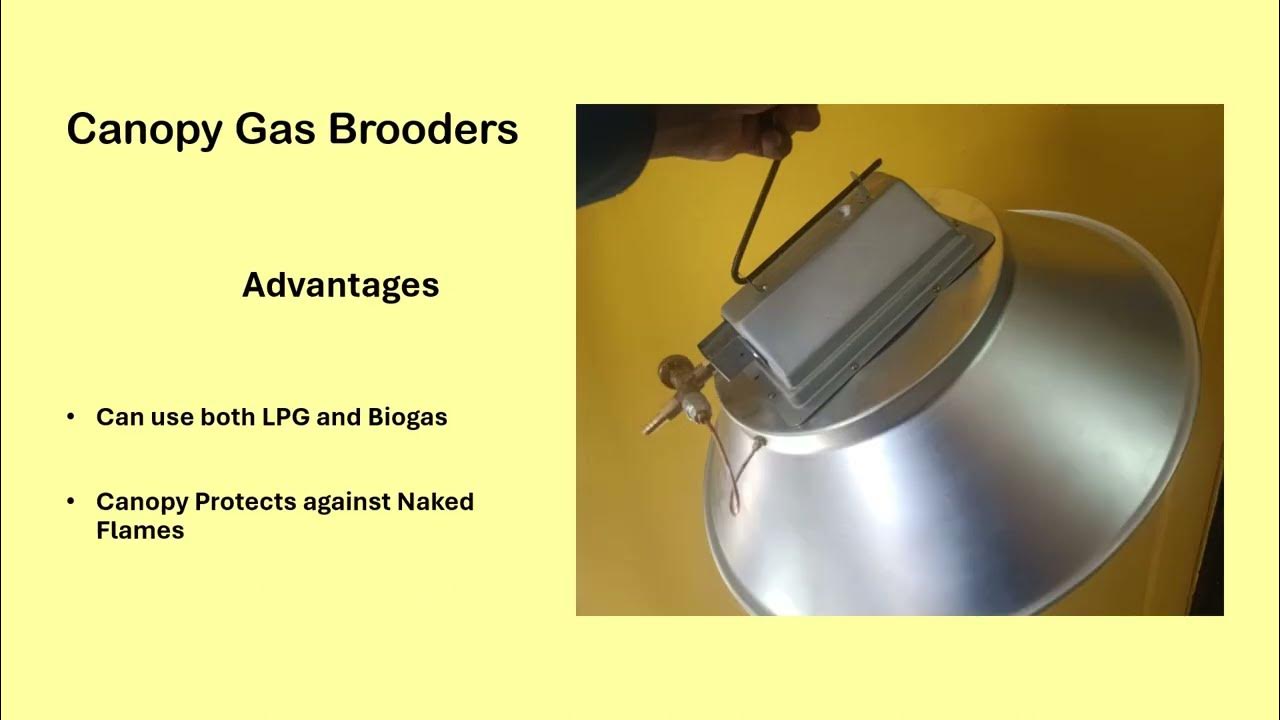This image depicts an informational poster with a bright yellow background. The black text on the left side reads "Canopy Gas Brooders" at the top, followed by the headline "Advantages." Below that are two bullet points: "Can use both LPG and biogas" and "Canopy protects against naked flames." The text is spaced out and positioned about 60% down the page.

On the right side of the poster, there is an image of a silver, dome-shaped device resembling a floodlight or heat lamp, angled around the five o'clock position. The device has an electrical box and a wire extending to the upper left corner. A hand, appearing to be male, is holding the device from behind with a black handle. The device's appearance includes a nozzle at the bottom which connects to a gas source. The background of the image and the poster itself is a consistent, bright yellow, providing a stark contrast to the black text and the silver device. The simplicity and clarity of the layout suggest it is an advertisement or informational piece related to gas heating equipment.